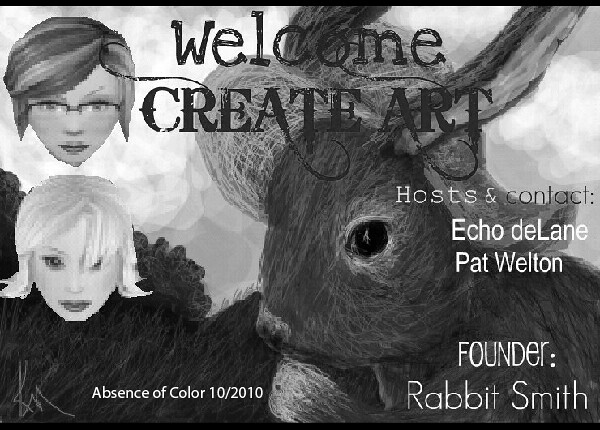This black and white advertisement promotes an art event titled "Welcome, Create Art." Dominating the left side of the image are the pixelated portraits of two women stacked vertically—one with dark, short hair and black-rimmed sunglasses, and the other with blonde hair, red lipstick, and bangs. The right side features a hand-drawn rabbit wearing a straw gardening hat, holding a paw up to its mouth. This whimsical background, possibly depicting an outdoor scene with a grassy field and sky, is dark and pixelated, giving a unique aesthetic. In white text on the right, it lists the hosts: Echo Delane and Pat Walton, and mentions the founder, Rabbit Smith. At the bottom left, it states, “Absence of Color, 10/2010.”